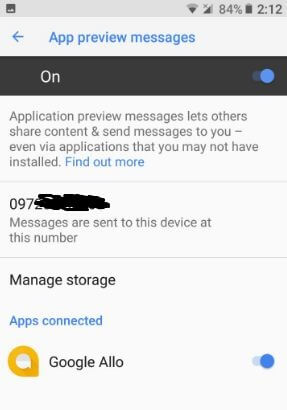The image on the smartphone screen captures a settings interface specifically related to app preview messages. The settings panel, set against a grey background, shows that app preview messages are enabled. The description below reads: "Application preview messages let others share content and send messages to you. Often via applications that you may not have installed." A hyperlink labeled "Find out more" is available for further information.

Beneath this text, a phone number is partially obscured with a black scribble, ensuring privacy. The text following the obscured number states: "Messages are sent to this device at this number."

Further down, a section titled "Manage storage" lists connected apps, with Google Allo shown as enabled.

At the very top-right corner of the smartphone screen, icons display the communication signal strength, Wi-Fi signal strength, a battery indicator showing 84% remaining, and the current time, 2:12.